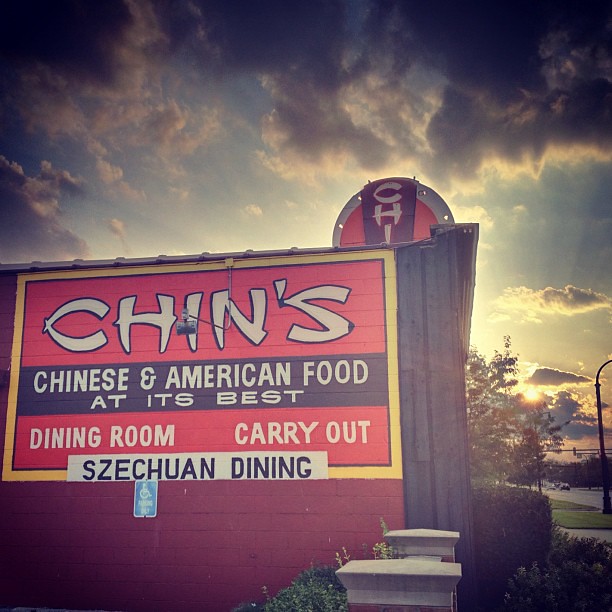This photograph captures an outdoor scene featuring a prominent sign for "Chin's," a Chinese and American restaurant. The sign, a combination of wood and brick, prominently displays in large white letters: "Chin's," followed by "Chinese and American food at its best," "Dining room," "Carry out," and "Szechuan Dining." Below these inscriptions, a handicap parking sign is visible on the brick base. To the right and foreground, the sign is bordered by white columns possibly forming part of a bench, set against a backdrop of lush grass, shrubs, hedges, and trees. 

The sky, vivid with shades of blue and white clouds, suggests it is either late afternoon or early evening, adding a warm glow to the scene. Above the main sign, partially obscured by its positioning, is a circular sign reading "Chai," hinting at another establishment or offering.

The overall photograph exhibits a heavy vignette with a notable purple hue, likely due to an applied filter, which adds an unusual contrast to the image.